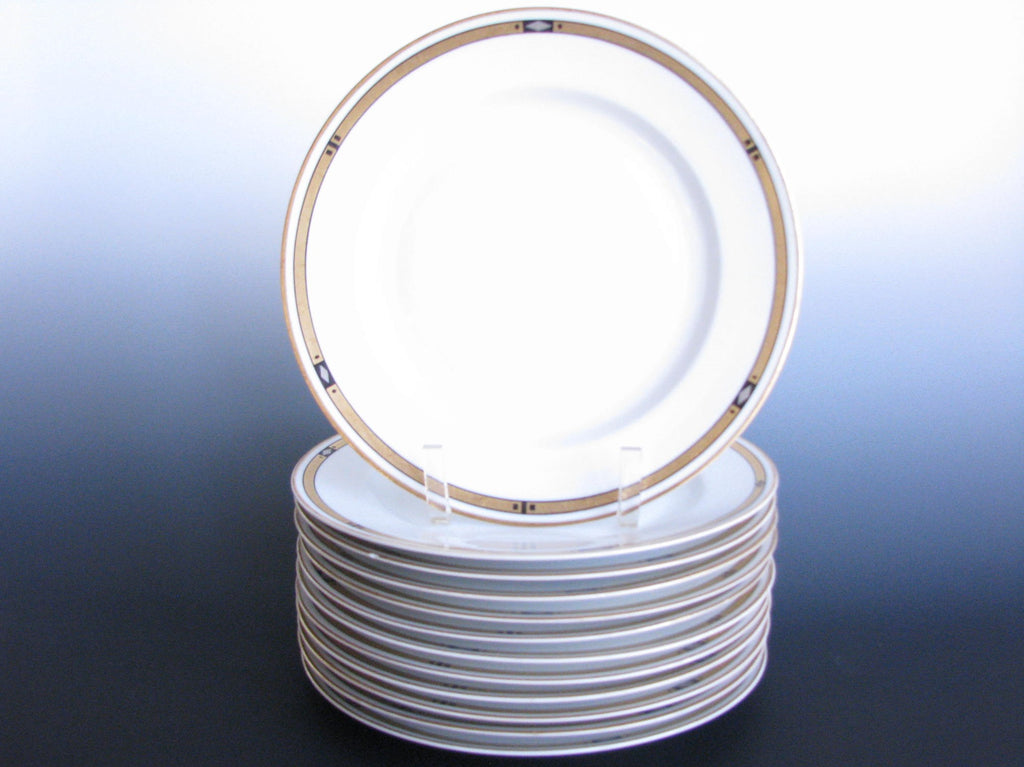The image showcases a set of white plates, prominently displayed against a gradient background that transitions from dark blue at the bottom to lighter blue and almost white at the top. The plates are accentuated with a gold trim that features intricate black and gray diamond patterns. There are approximately 10 to 11 plates neatly stacked one on top of the other. At the top of the stack, one plate is positioned upright, held in place by clear, translucent stands to display its detailed design to viewers. The lighting highlights the plates, casting a subtle shadow at their base and enhancing their elegant features, making it suitable for a sale listing.